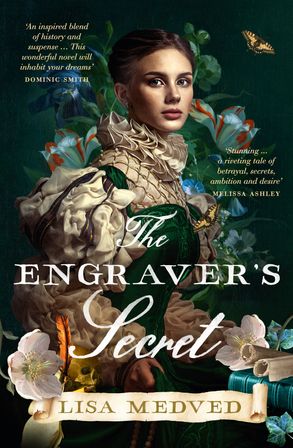The cover of the book features a detailed and enchanting illustration of a young woman in an elaborate green and tan dress with intricate white details, including white sleeves. Her short brown hair complements the elegant setting. She appears to be seated amidst a lush background filled with vibrant flowers and leaves in green, red, and white tones, along with the subtle presence of a yellow butterfly in the upper right corner. The image exudes a historical and enigmatic vibe, emphasizing elements of nature and grace.

Prominently displayed in the center of the image is the book's title, "The Engraver's Secret," in white lettering, with "The" and "Secret" in cursive script and "Engraver's" in a serif font. At the bottom, the author's name, Lisa Medved, is elegantly written in gold letters on a scroll-like banner. Two quotes adorn the image: one in the upper left corner, stating, "An inspired blend of history and suspense, this wonderful novel will inhabit your dreams," attributed to Dominick Smith, and another on the upper right, reading, "Stunning. A riveting tale of betrayal, secrets, ambition, and desire," by Melissa Ashley. The cohesive design and intricate details collectively create an invitation into a world of mystery and elegance.